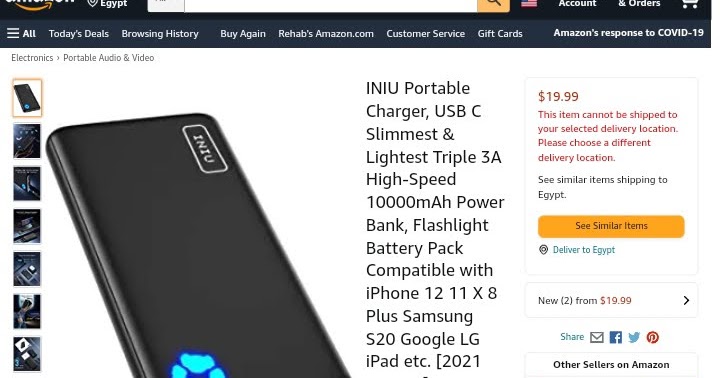A screenshot of an Amazon order page featuring a portable charger from the brand INIU. The charger is compatible with various devices including the iPhone 12, 11, and 8 Plus, as well as Samsung S20, Google LG, and iPads. The product is a USB-C type, marketed as the slimmest and lightest triple 3A high-speed 10,000mAh power bank with an integrated flashlight. The visible portion of the product title ends with "2021," and the item is priced at $19.99. Below the price, a message in red text alerts that the item cannot be shipped to the selected delivery location, advising to choose a different one. Additionally, there is a prompt in black text to "see similar items shipping to Egypt," accompanied by an orange button labeled "See similar items."